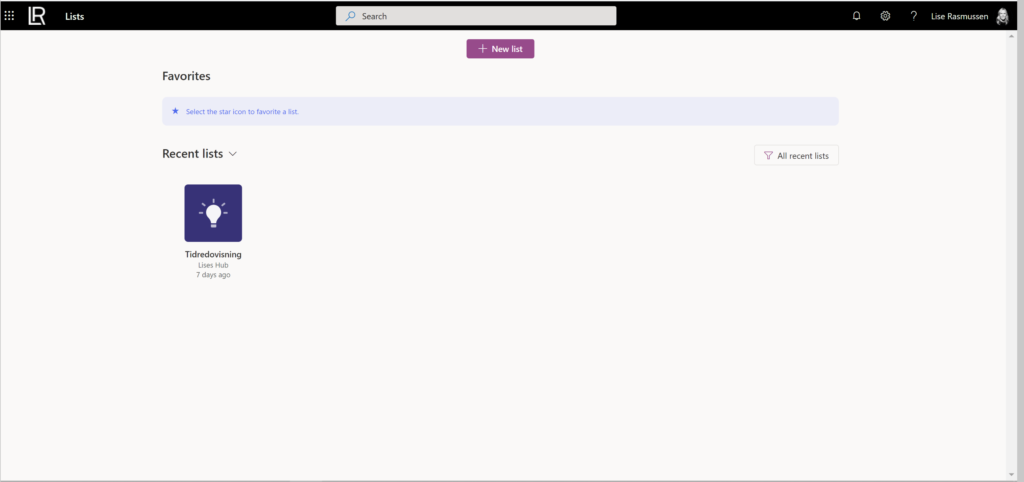The image appears to be a screenshot from a website, possibly related to user-generated lists or content organization. At the top of the page, there are several clickable menu items, including "Lists," a notifications tab, a settings tab, and a help or information tab marked with a question mark. The user profile displayed is named "Lise Rasmussen," and next to the name, there is a small thumbnail image, which seems to depict a girl, although the facial details are unclear.

Just below the top menu, there is a search bar for navigating the site. An option to "Add New List" is prominently displayed beneath the search bar. On the sidebar to the left, sections are labeled, including "Favorites," with instructions to select a star icon to favorite a list, and "Recent Lists," accompanied by a filter dropdown menu that defaults to "All Recent Lists."

In the "Recent Lists" section, only one entry is shown. The list is titled "Tiedre Dovzing," identified by an icon of a lit light bulb against a purple background. Subtext indicates that this list is part of "Lise's Hub" and was created seven days ago.

The remainder of the screen is mostly white, with no additional content or features visible beyond those already described.